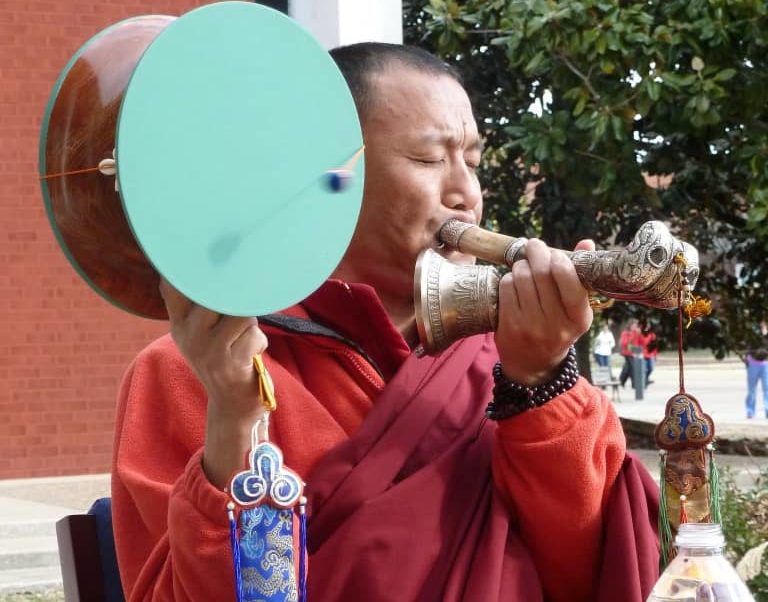The image features a man of Asian descent, possibly a Buddhist monk, deeply immersed in a ceremonial act. He is adorned in a striking red robe, eyes closed in concentration. In his left hand, he holds a pipe-like musical instrument, which appears to be crafted from wood or bone, embellished with some ornate gold metal. This instrument is brown with grayish hues and has a red charm hanging from its end. Additionally, in the same hand, he delicately grasps a golden bell, adorned with intricate designs. His right hand supports a unique percussion instrument, blue at the base and wooden in the middle, featuring two sides and strings with beads or shells that create sound when spun. A black bracelet adorns his left wrist, adding to the detailed narrative of his attire. The backdrop reveals a green tree and a brick building on the left, suggesting a summertime setting with a few people dispersed under the tree, adding context to this ceremonial snapshot.